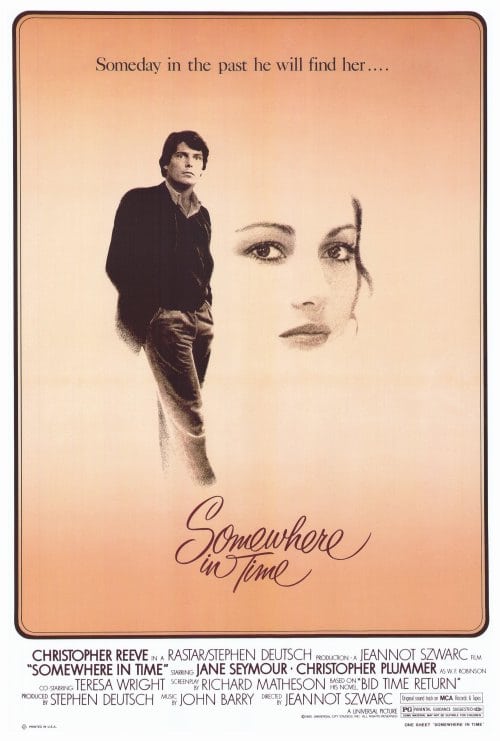The image is a vintage movie poster for the classic film "Somewhere in Time," starring Christopher Reeve. Dominating the poster is a soft, neutral-toned background blending beige and white, with hints of light gold and bronze. At the center-right of the poster, we see the slightly distraught face of a woman, while to her left stands a man, presumably Christopher Reeve, dressed in a black jacket with his hands in his pockets, staring off neutrally into the distance. The title "Somewhere in Time" is elegantly scripted in cursive at the bottom. Above, the tagline "Someday in the past, he will find her" is prominently displayed in black text. The lower portion of the poster includes credits for the cast and crew as well as the movie's PG rating. The film's plot centers around Reeve's character, who learns to time travel through intense concentration, goes back in time, falls in love, but is tragically pulled back to his original time, unable to return.